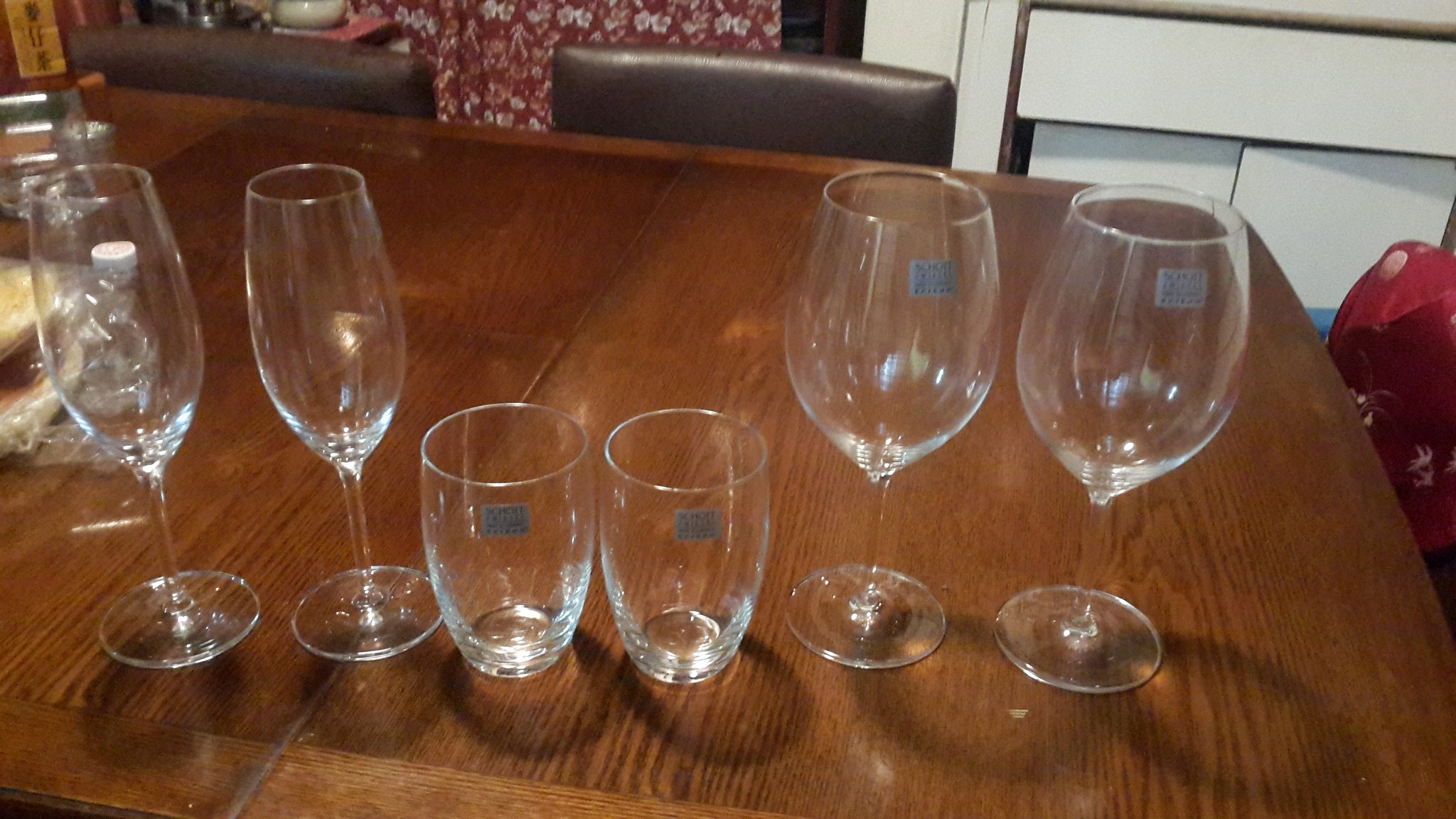The image depicts a wooden dining table with various types of empty glasses neatly arranged on it. There are three distinct sets of glasses, each consisting of two pieces. On the left side, the first set includes two champagne-type glasses with slender stems, followed by a pair of shorter, stemless glasses that are U-shaped and reach about halfway up the height of the champagne glasses. These glasses feature a blue sticker on their fronts. The final set on the right comprises standard wine glasses with shorter stems, also adorned with blue stickers. In the background, we see two brown leather chairs pushed into the table and a mix of hanging red fabric and white cabinets or drawers along the wall. A bottle and some other small objects are positioned on the far left of the table.